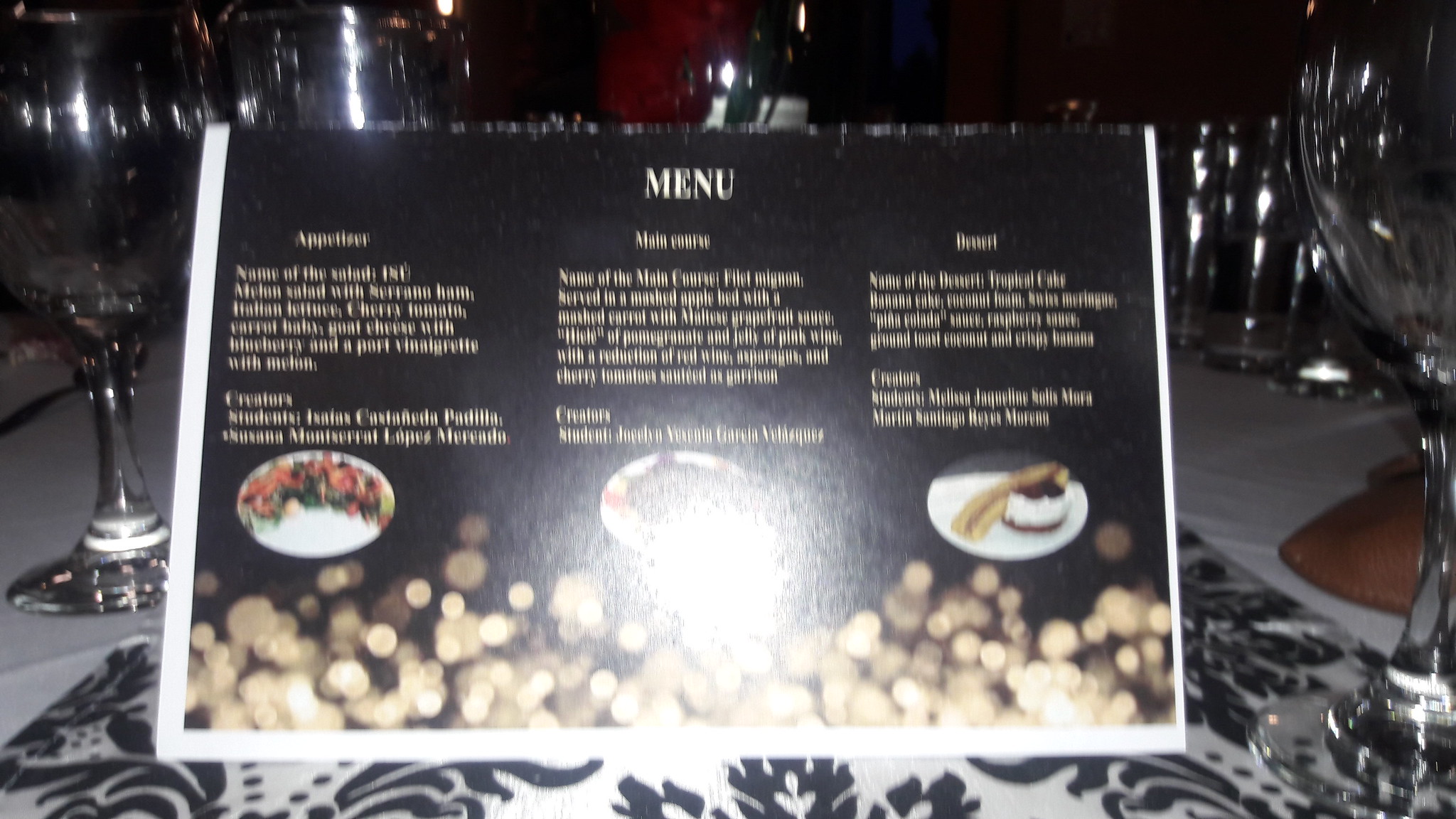This photo, taken in a dimly lit restaurant, captures an elegantly set table with a prominently displayed menu. The table is adorned with a white table runner featuring black leaf and flower motifs interspersed with dotted patterns. The menu, though too blurry to read in its entirety due to the dim lighting and bright glare in the middle, lists appetizers, main courses, and possibly desserts. 

In the background, clear wine glasses and cylindrical glasses are arranged neatly, with three visible wine glasses and several smaller glasses. A clear wine bottle with a visible label is situated near the top of the menu, suggesting someone may be holding it. Additionally, a subtle peach-colored blur suggests the presence of a person in the background, adding to the lively ambiance of the scene.